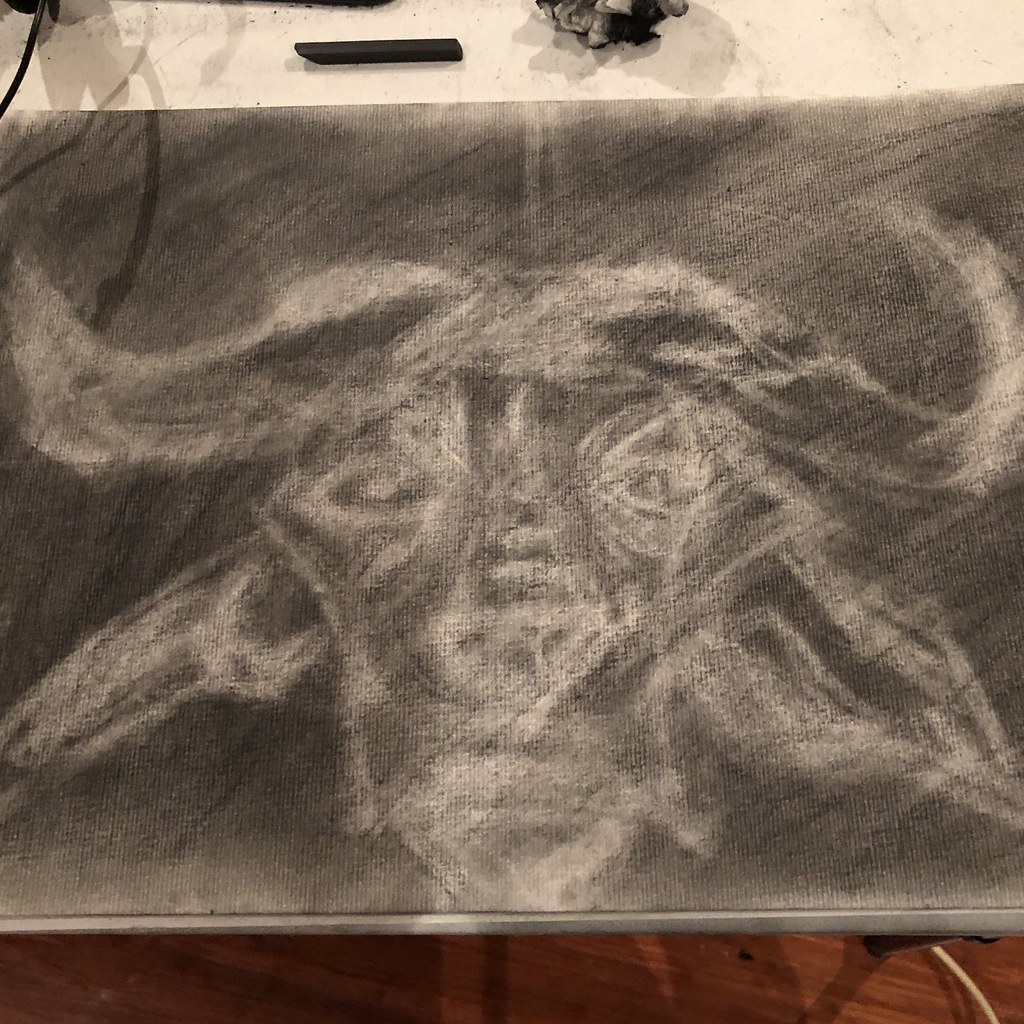In this charcoal drawing, the artist has depicted a powerful bull with prominent horns extending from both sides of its head. The detailed artwork fills the majority of the canvas, conveying a sense of motion and strength. At the top of the image, a piece of charcoal rests on the surface, hinting at the medium used. Towards the upper center, a rag or paper towel is visible, likely employed for blending and shading. The drawing seems to be positioned on a table, as indicated by the visible support leg peeking from below. The floor beneath the table has a rich cherry wood varnish, adding warmth to the setting. The entire scene exudes an atmosphere of an artist's workspace, filled with tools of creation and the vibrant energy of the creative process.